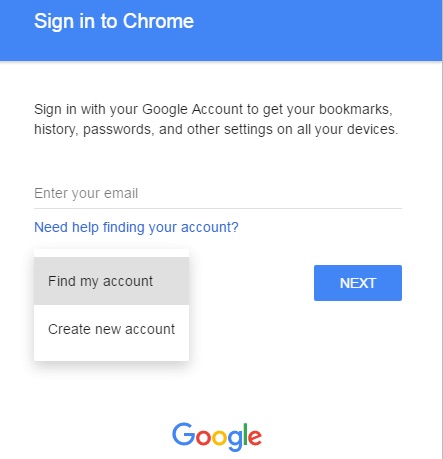The image depicts a user interface designed for signing into Chrome. The layout is slightly taller than it is wide, with a blue bar at the top occupying approximately 10-15% of the image's height. This blue bar features left-aligned, white text that reads "Sign into Chrome."

Below the blue bar is a small white gap, contributing to the predominantly white background of the image. Centered text below this gap, slightly indented from both the right and left margins, is written in black and states: "Sign in with your Google account to get your bookmarks, history, passwords, and other settings on all your devices."

Following another white space, there's a prompt in light gray text saying "Enter your email," accompanied by a gray underline, indicating where users can input their email address. 

Directly below this input area, blue text identical in hue to the top bar reads "Need help finding your account?" 

In the bottom left section of the image are two horizontal rectangular buttons stacked vertically. The top button, with a medium gray background, reads "Find my account" in black text. The button below it has a white background and says "Create new account," also in black text. 

To the right of these buttons, aligned to the right-hand side of the image, is another horizontal rectangle filled with the same blue color as the top bar. It contains the white text "Next" centered within.